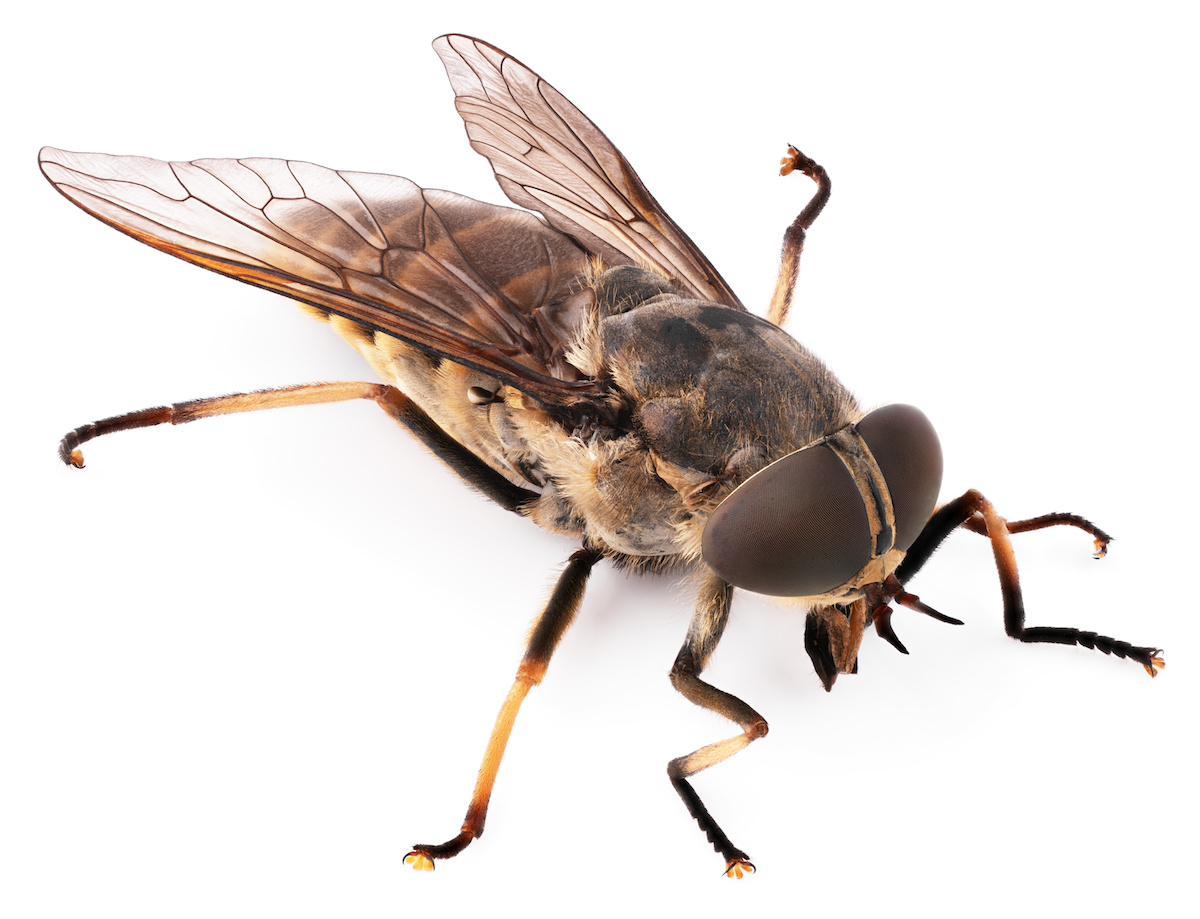This is an extremely detailed, zoomed-in photograph of a fly set against a stark white background. The entire fly is visible in the image, showcasing its distinctive features in stunning clarity. The most prominent characteristic is its large, brown eyes that dominate its head, which is divided by a dark brown vertical strip. Behind these imposing eyes, a shell-like structure can be observed, adding to the intricate detail. 

The fly's body exhibits a complex color scheme of dark brown, black, and patches of a yellow hue that almost blend into brown, giving it a subtle gradient effect. It possesses six legs, three on each side, all oriented towards the lower right part of the image. The transparent wings, tinted with dark brown patterns, are another focal point, highlighting the delicate yet robust structure of the insect's anatomy. Additionally, two sharp fangs protrude from its mouth area, adding to the characteristic features that define its predatory nature.

Despite some debate over whether it could be a moth, the photograph distinctly captures the essence of a fly, albeit with some unusual textured hair which contributes to its unique appearance in this close-up presentation.